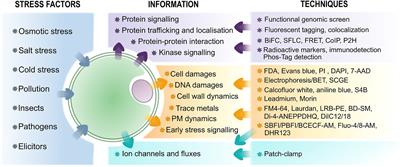This informational diagram is centered around a perfectly spherical, green cell with an olive-shaped purple segment on its right side. It features multiple arrows leading to and from various sections, each with colored backgrounds and bullet points describing different aspects.

On the left, a blue section labeled "Stress Factors" lists: osmotic stress, salt stress, cold stress, pollution, insects, pathogens, and elicitors, with arrows pointing into the cell. Adjacent to it, the gold-colored "Information" section has arrows leading out from the cell and includes bullet points such as cell damages, DNA damages, cell wall dynamics, trace metals, PM dynamics, and early stress signaling.

Following that, an adjacent turquoise section labeled "Information" holds a single bullet point, ion channels and fluxes, with turquoise arrows leading both in and out of the cell. Below these, another turquoise arrow points to a "Techniques" section, which lists patch clamp.

A purple section labeled "Information" includes arrows leading out from the cell, detailing protein signaling, protein trafficking and localization, protein-protein interaction, and kinase signaling. Another purple box labeled "Techniques" points to this and lists methods including functional genomic screen, fluorescent tagging, colocalization, BIFC, SFLC, FRET, CO-IP, P2H, radioactive markers, immunodetection, and FOS tag detection.

Finally, a yellow section titled "Techniques," linked to the gold "Information" section, mentions FDA, Evans blue, PI, DAPI, 7AAD, electrophoresis, BET, SCGE, calcofluor white, aniline blue, S4B, leadmium, morin, FM464, Lourdan, LRBPE, BOSM, DI-4-ANE, PPE, DHQ, DISC-1218, SBFI, PBFI, BCECFAM, FLUO-4-8-AM, and DHR123.

Overall, the diagram visually organizes stress factors, cellular responses, and the techniques used to study these biological processes.